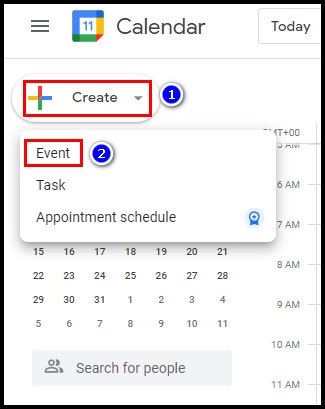The screenshot of a Google Calendar interface is captured in a rectangular shape with a thin black border encompassing it on all four edges. The predominant background color is white. In the very top left corner, there are three horizontal black lines arranged vertically. Adjacent to them on the right is a square composed of a blue top and left border, a yellow right border, and a green bottom border. Within this square is a white box featuring blue text that reads "11."

To the right of this square, in the central top area of the image, is the black text "Calendar." At the top right corner, there is a white rectangular button with a thin gray border, containing black text that states "Today." Beneath this text, a single long light gray line spans horizontally from the left to the right, forming a header or divider.

Below this horizontal line, the white background resumes. An oval-shaped button labeled "Create" appears in black text, which is prominently highlighted by a red rectangular outline, drawing attention to this section. Further down, a white rectangular box displays the options "Event," "Task," and "Appointment Schedule" in black text.